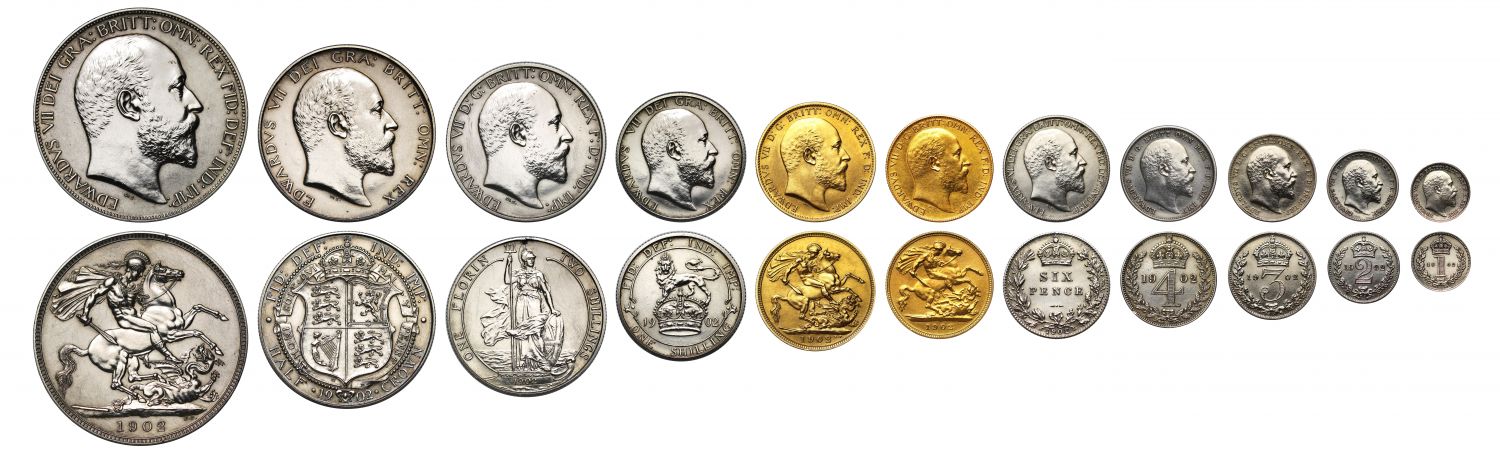This image displays a collection of old British coins arranged in two rows, with each row consisting of 12 sets. Each set includes the front and back of a coin. The fronts, predominantly silver save for two gold coins in the center, consistently display the face of a bald man with some hair on the sides, a beard, and a mustache. The backs vary significantly, featuring designs such as a man riding a horse, an emblem, and other intricate patterns. The coins are organized by size, starting with the largest on the left and gradually decreasing in size as one moves to the right. The arrangement further illustrates a historical progression, possibly showing different denominations, which might range from one pence upwards.